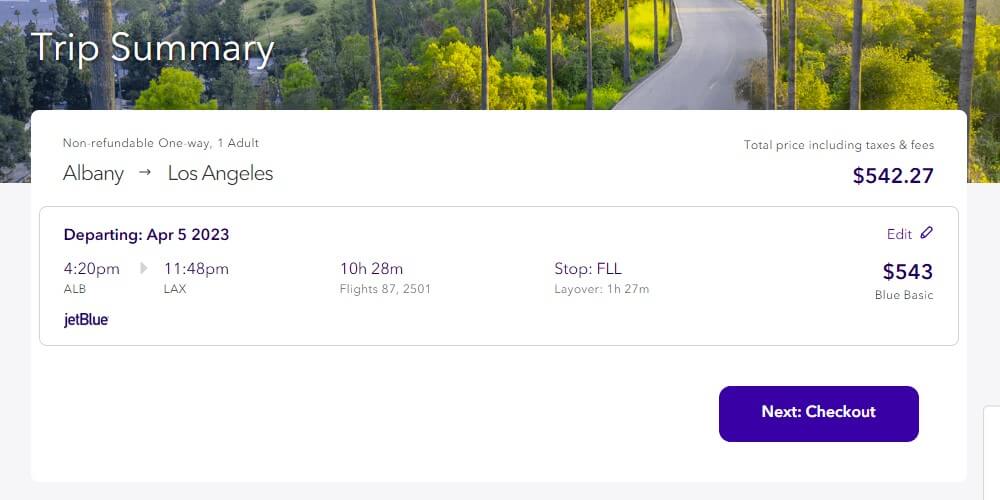**Detailed Caption:**

The screenshot captures the details page of an individual's planned trip from Albany to Los Angeles. At the top of the image, the words "Trip Summary" are prominently displayed in white font against a scenic forest background. This background features a winding gray road cutting through lush, green vegetation with bushes and trees lining both sides. To the left side of the image, a small body of water is faintly visible, adding to the vibrant and lively ambiance, with shades of yellow-green near the road and more muted greens towards the edges.

Central to the screenshot is a rounded rectangular panel highlighting key trip details. It specifies that the ticket is non-refundable and for an adult, with the total price, including taxes and fees, noted as $542.27 in a purple font. The itinerary lists the journey from Albany to Los Angeles.

Below this information, another rounded rectangular outline details the flight specifics. It states that the departure from Albany is scheduled for April 5th, 2023, at 4:20 PM, with an expected arrival at LAX (Los Angeles) at 11:48 PM. The total travel time is 10 hours and 28 minutes, and it includes a stop at FLL (Fort Lauderdale) with a layover time of 1 hour and 27 minutes. Further details in gray font mention the flight numbers as 87 and 2501. The fare class mentioned is "Blue Basic," and it is clarified that the airline for this journey is JetBlue.

At the bottom of the panel, there is another rounded rectangular button in purple with the word "Checkout" in white font, inviting the user to complete the transaction.